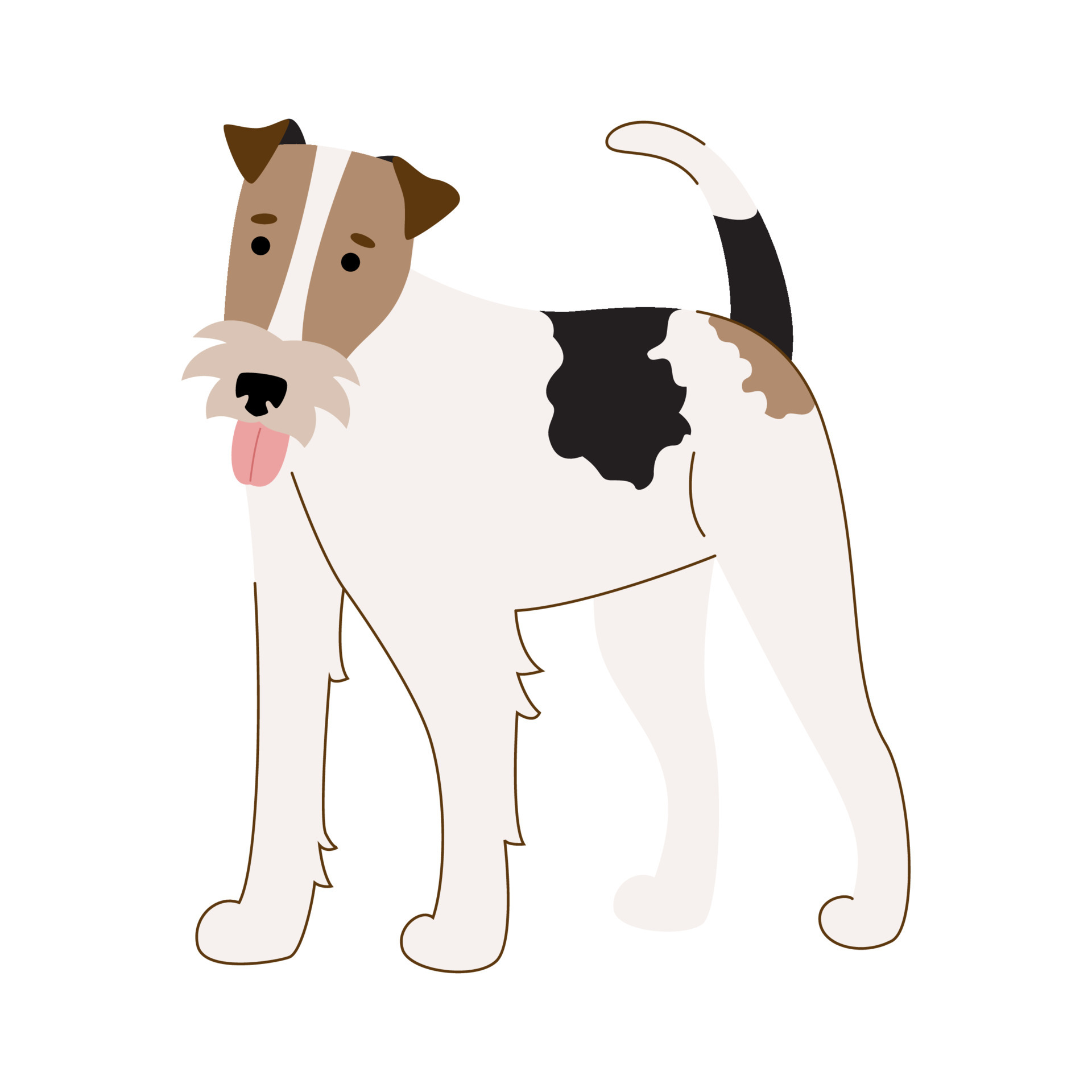This is a detailed cartoon illustration of a medium-sized dog with a predominantly white body featuring distinct patches and intricate details. The dog appears on a pure white background, outlined with a dark brown thin line that highlights its form. It has tall and notably long legs, with the front two legs fully outlined, while only the far right side of the rear right leg is outlined from our perspective.

The dog's back showcases an irregular black splotch, while a light brown patch adorns its rear end. Protruding from behind this brown splotch, the tail is striped with black at the bottom and the same eggshell white at the top. The head of the dog is mostly light brown on either side, with a prominent white stripe running down the middle from the top of its head to its snout. This stripe compliments its dark brown, triangular ears which have black underneath.

The dog's face exudes character with black, perfectly circular eyes set within the brown portions of its face, each eye topped with a dark brown oval eyebrow. Positioned below the eyes is a quaint beige beard with three distinct points on either side. The nose is black, and a pink tongue with a red line through the middle hangs down from the mouth, giving a friendly and approachable vibe. Overall, the illustration suggests the dog as a charming and potentially lovable main character, fitting seamlessly into a children's book.